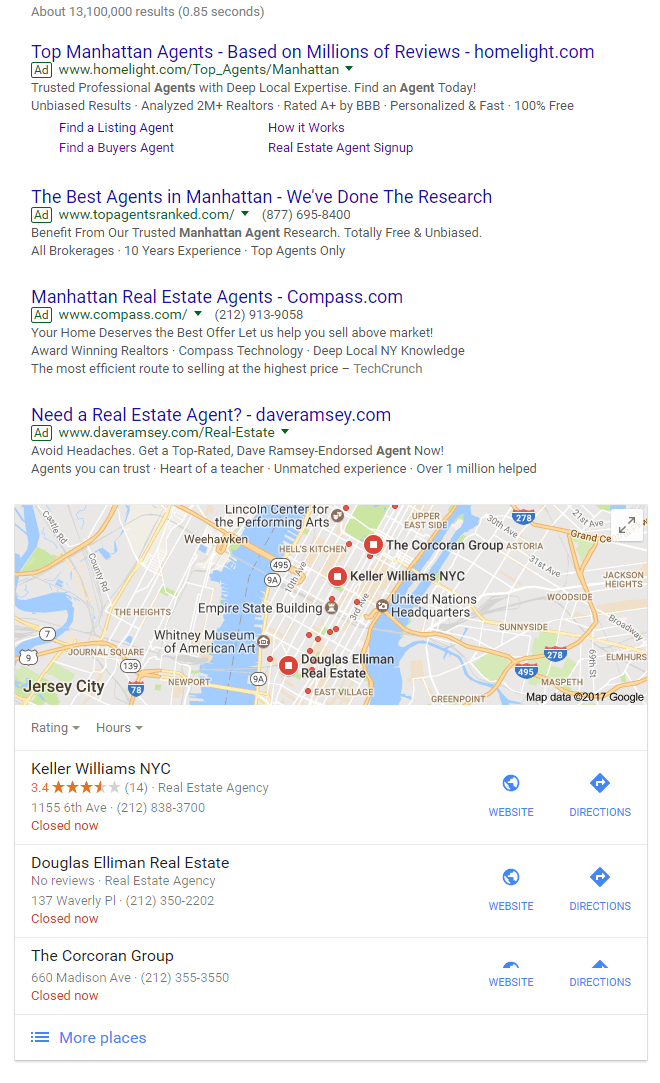**Caption:**

A detailed view of a webpage, showcasing a white background and a search results summary at the top left, indicating "about 13,100,000 results (0.85 seconds)." Below this, an advertisement for HomeLight is prominently displayed. The ad promotes "top Manhattan agents based on millions of reviews" and lists the website URL "www.homelite.com/top_agent/manhattan." An arrow points downward towards the ad text, which highlights features such as "trusted professionals, agents with deep local expertise," along with a call to action to "Find an agent today!" The ad emphasizes unbiased results, the analysis of over 2 million realtors, an A+ rating (presumably by the BBB or another agency), and the promise of personalized, fast, and 100% free service.

Further down, the ad provides options to "Find a listing agent," "Find a buyer's agent," and a link for real estate agents to sign up. A "How it works" section is also mentioned, offering prospective users guidance on navigating the services provided.